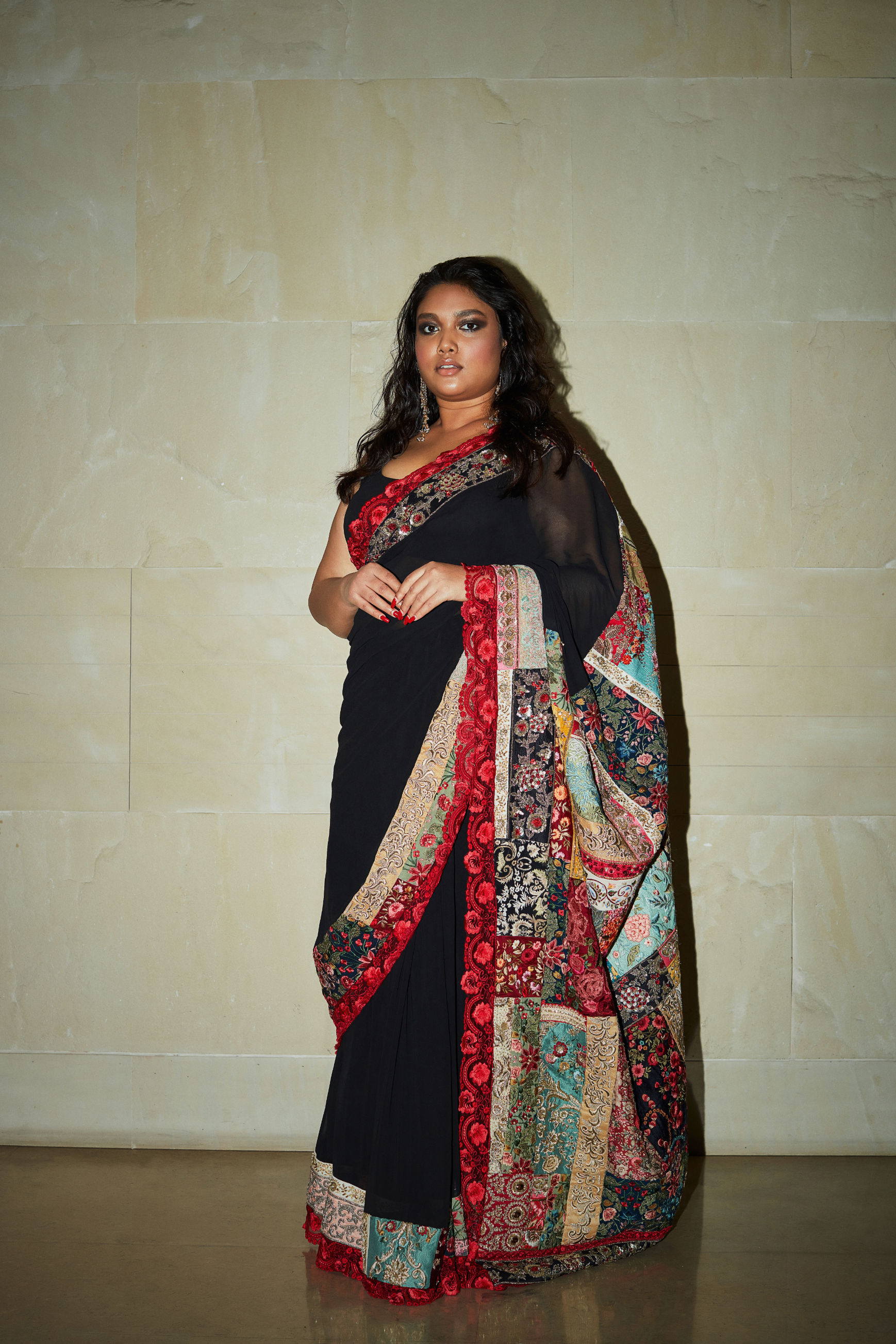The image features a woman standing in the center of the frame, gazing directly at the camera with an assured pose. She has tan skin and long, shoulder-length, dark curly hair. She is adorned in a striking, ornate black dress that showcases a rich cultural influence. The dress has an intricate design with bright patterns, particularly at the neckline and the edges. Her right arm is sleeveless, while her left arm has a long black sleeve and is seen holding a colorful sash draped across her back. The sash, made of satin, boasts a red border and a patchwork of vibrant colors including reds, turquoises, beiges, blacks, and pinks. It complements the dress beautifully, which also features a red-bordered hem with decorative patterns at the bottom. The woman's nails are painted red, adding a touch of detail. She is accessorized with long earrings that reach down to her neck. The background presents a white-yellowish wall and a brown floor, in a brightly lit setting which highlights the clarity and vividness of the image.